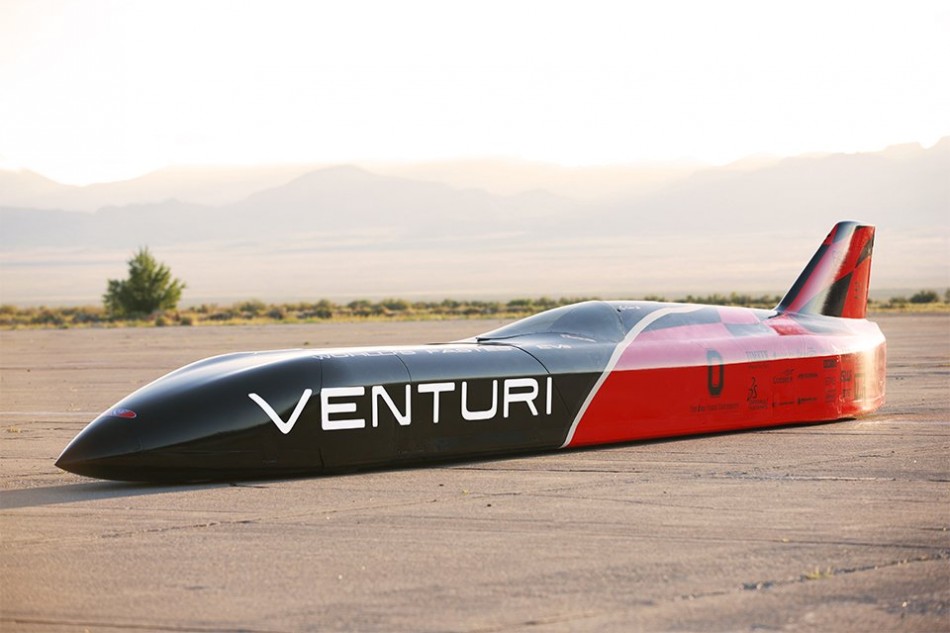This photograph captures a sleek, unusual vehicle that vaguely resembles a wingless jet or missile, positioned on a grey paved surface. The contraption, identifiable by the white text "Venturi" on its black nose and "Zero" on the adjacent red section, features a sharp front that slopes into a slightly elevated black cockpit. The vehicle is bisected by a white stripe, which separates the black front end from the vibrant red rear. At the back, a black and white fin protrudes. Surrounding the pavement is a strip of greenery with a single green bush on the left. The blurry backdrop reveals a hazy grey mountain range beneath a bright white sky.